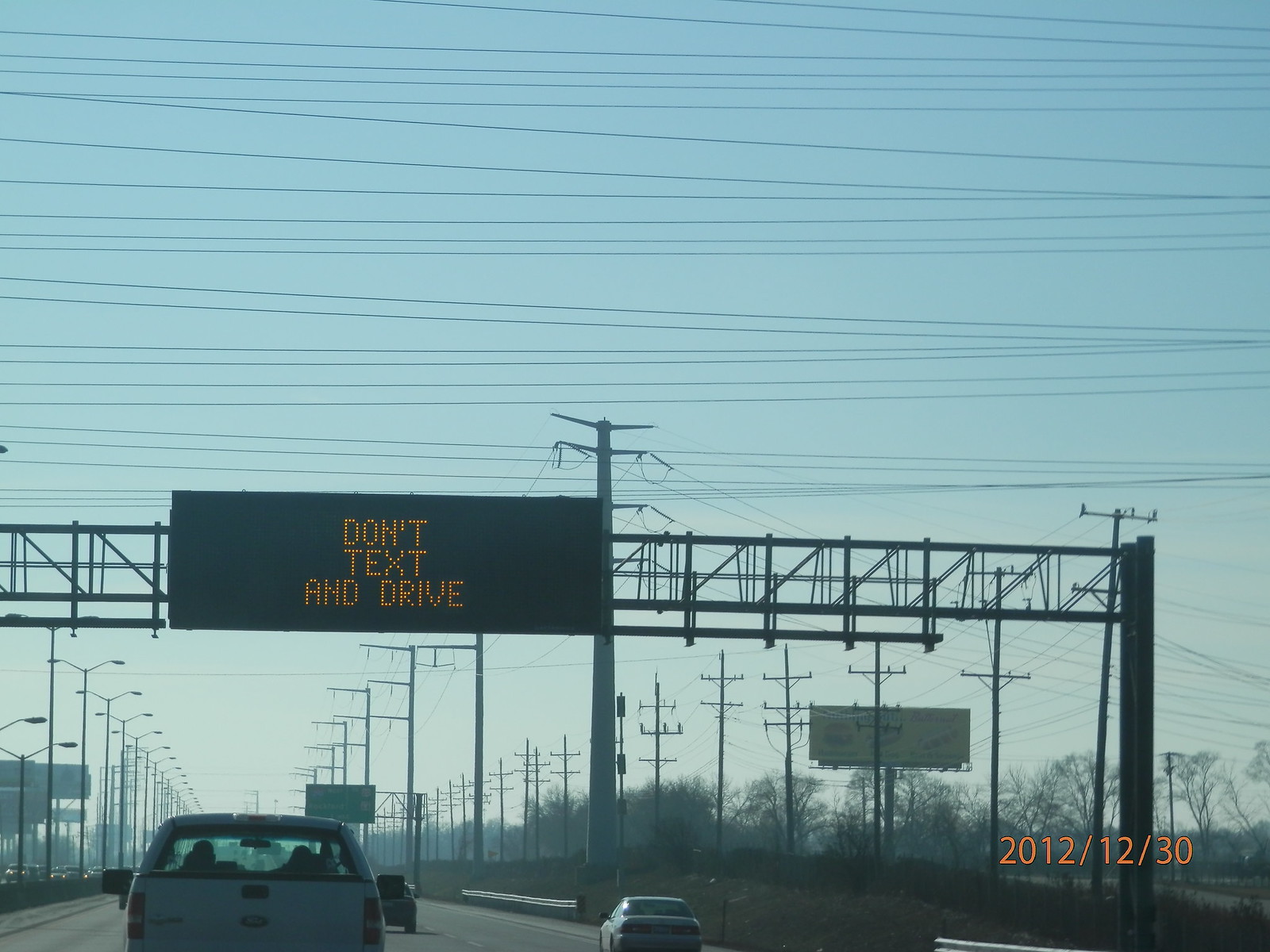The colour photograph captured outdoors from the perspective of a passenger or driver in a vehicle on a motorway in the United Kingdom showcases a typical scene heightened by specific details. Dominating the view from the vehicle’s windshield is a large raised gantry crossing the motorway lanes. This structure supports an electronic sign with illuminated orange letters that display the message, "Don't text and drive." The date stamp "2012/12/30" is visible in small orange text at the bottom right corner, indicating the photograph was taken in late December 2012. 

The motorway consists of several lanes with noticeable traffic. Directly ahead is a white vehicle, and beside it to the right, a small gray sedan is visible, followed by another car in the adjacent lane to the left. Lining the side of the road are rows of lampposts on the left and telegraph poles with crisscrossing wires on the right. Additionally, the scene includes glimpses of a grassy area at the lower right and trees without leaves in the distance, hinting at the season. The sky above is light blue and slightly cloudy, adding to the muted winter atmosphere.